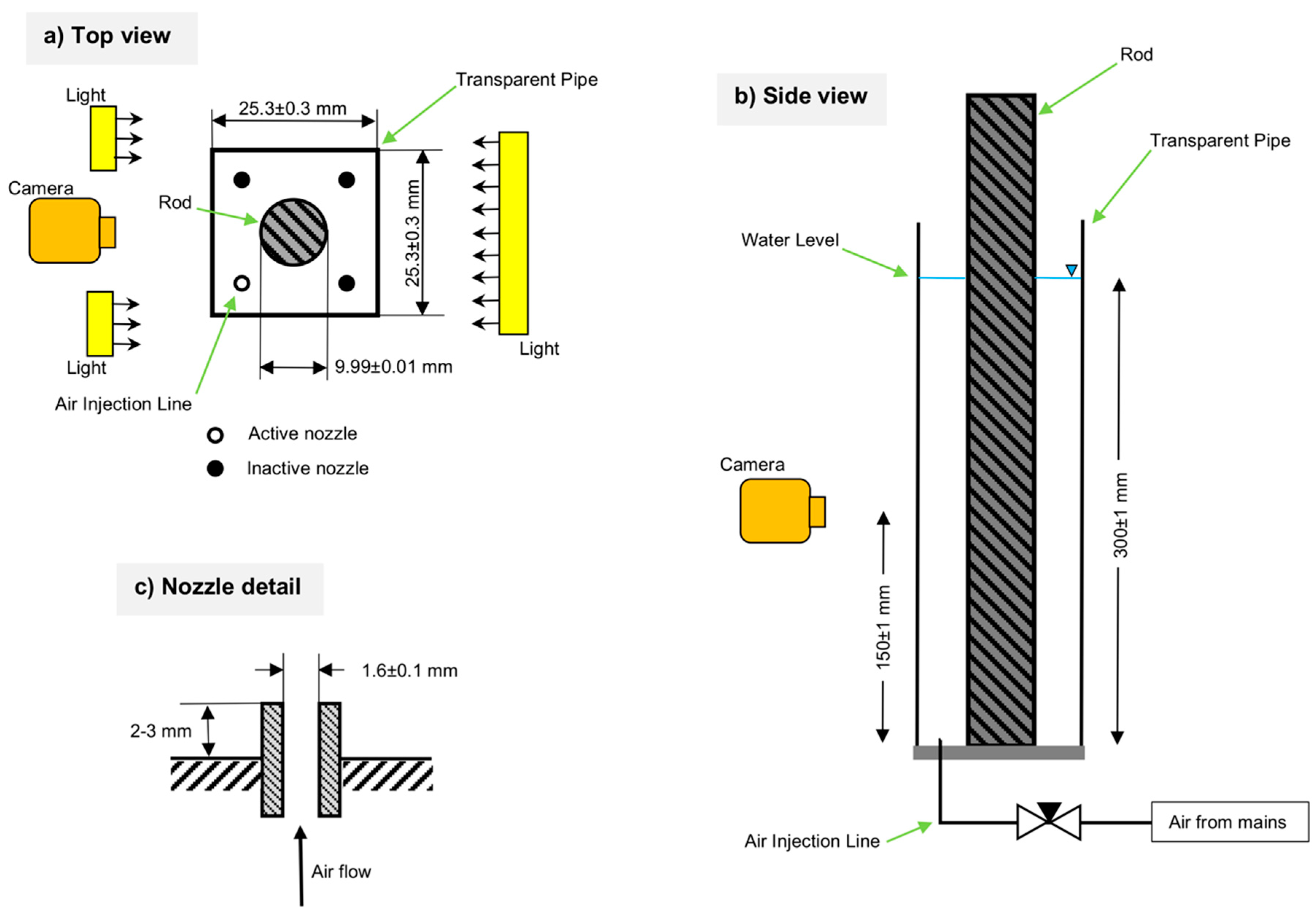This textbook-like schematic image, predominantly black and white with occasional color highlights, is divided into three parts: A (top view), B (side view), and C (nozzle detail). The top left section labeled "A top view" features a squared layout resembling a die with a large central circle adorned with gray and black stripes. To its right is a thin rectangular shape, while two smaller similar shapes are to its left, representing components labeled as light (yellow) and camera (orange). The central rod is also labeled. 

The right section labeled "B side view" displays a tall rectangular diagram, housing a camera, rod, light, transparent pipe, air injection line, and water level indicator. 

The bottom left corner, designated as "C nozzle detail," illustrates the finer points of the nozzle, focusing on airflow indicated by an upward arrow, and includes two measurements. Both the light and the camera labels are color-coded for clarity. The whole schematic is detailed with technical terminologies and labels, portraying a detailed and comprehensive technical design.